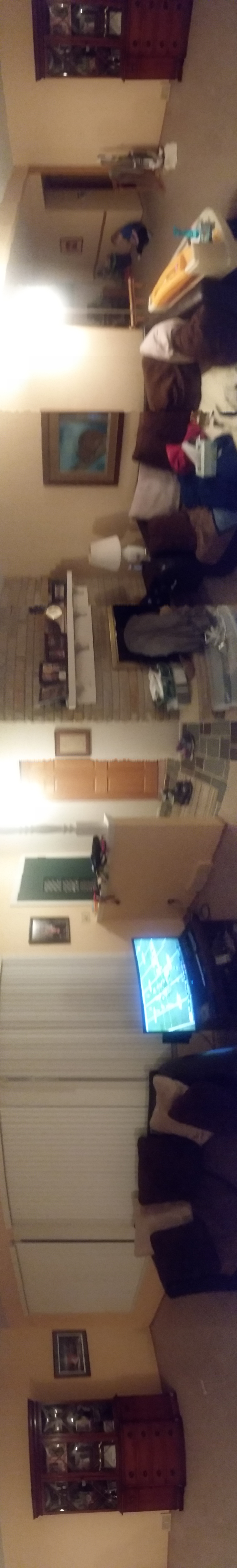A panoramic view of a cozy living room, captured in a long vertical image, showcases a warm and inviting interior. A laptop with a glowing screen rests open on a comfortable couch, hinting at a lived-in and tech-savvy space. The tan carpet complements the soft tan walls, which are adorned with various pieces of artwork. A shelf adorned with a clock and framed photos adds a personal touch to the decor. To the left of the image, an entertainment center or hutch displays an array of decorations and knickknacks, enhancing the room's homey ambiance. A door and lamp further frame the space, while the floor is scattered with various items, contributing to a somewhat cluttered yet charmingly authentic feel. The distant perspective of the photo makes it challenging to discern finer details, but the overall atmosphere is one of casual comfort and personalized style.